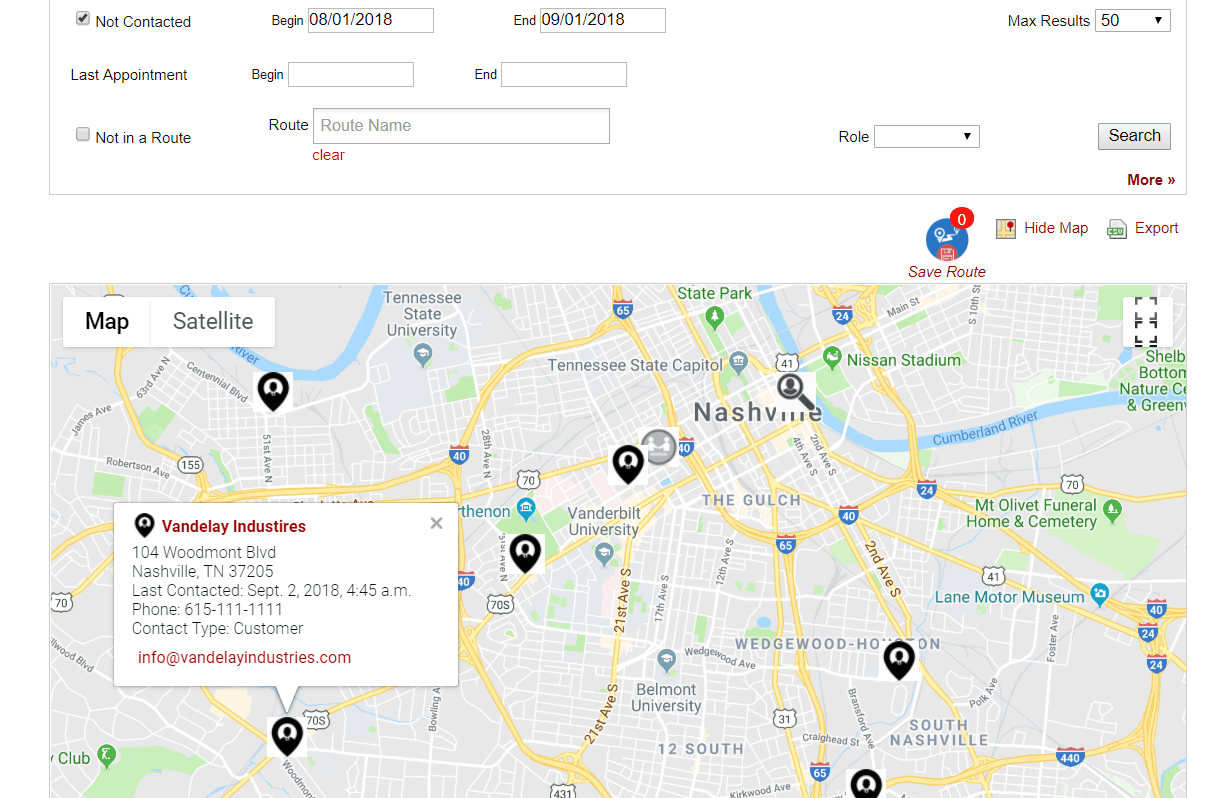Certainly! Here's a cleaned-up and highly detailed caption for the described image:

---

The image depicts a detailed interface of a digital form and map display. At the top of the form, there is a field with a white background bordered by a light gray line. In the top left corner of this field, it shows the status "Not Contacted" with a tick box that is checked with a black check mark. Moving towards the right, the form contains the word "Begin" in black lettering, followed by a rectangular field outlined in light gray, displaying the date "08/01/2018". To the right of this field, it says "End" next to another rectangular field with a light gray border, which shows the date "09/01/2018".

On the next line, the form reads "Last Appointment," followed by "Begin" and a fillable rectangular field. Towards the right, there is another fillable rectangular field with the label "End" adjacent to it. 

Further down, the form labels "Not in a Route" with an unchecked gray tick box to the left. Towards the right, the word "Route" is displayed in black, followed by an editable field titled "Route Name" in light gray text. Beneath this field, in small red lettering, it says "Clear." To the right, the label "Role" is shown alongside a drop-down menu, which currently has no selection. Further right, there is a gray "Search" button.

Directly beneath the "Search" button is a bold maroon option labeled "More," accompanied by two arrows pointing towards the right. Below this section, the image displays a large map.

On the lower left corner of the map, there is an overlay notification that reads "Vandelay Industries" with the address "104 Woodmont Boulevard, Nashville, Tennessee 37205." It also shows the last contact date as "September 2nd, 2018, 4:45 AM" and provides a phone number "615-111-1111".

---

This revised caption captures the detailed content and layout of the described image clearly and concisely.